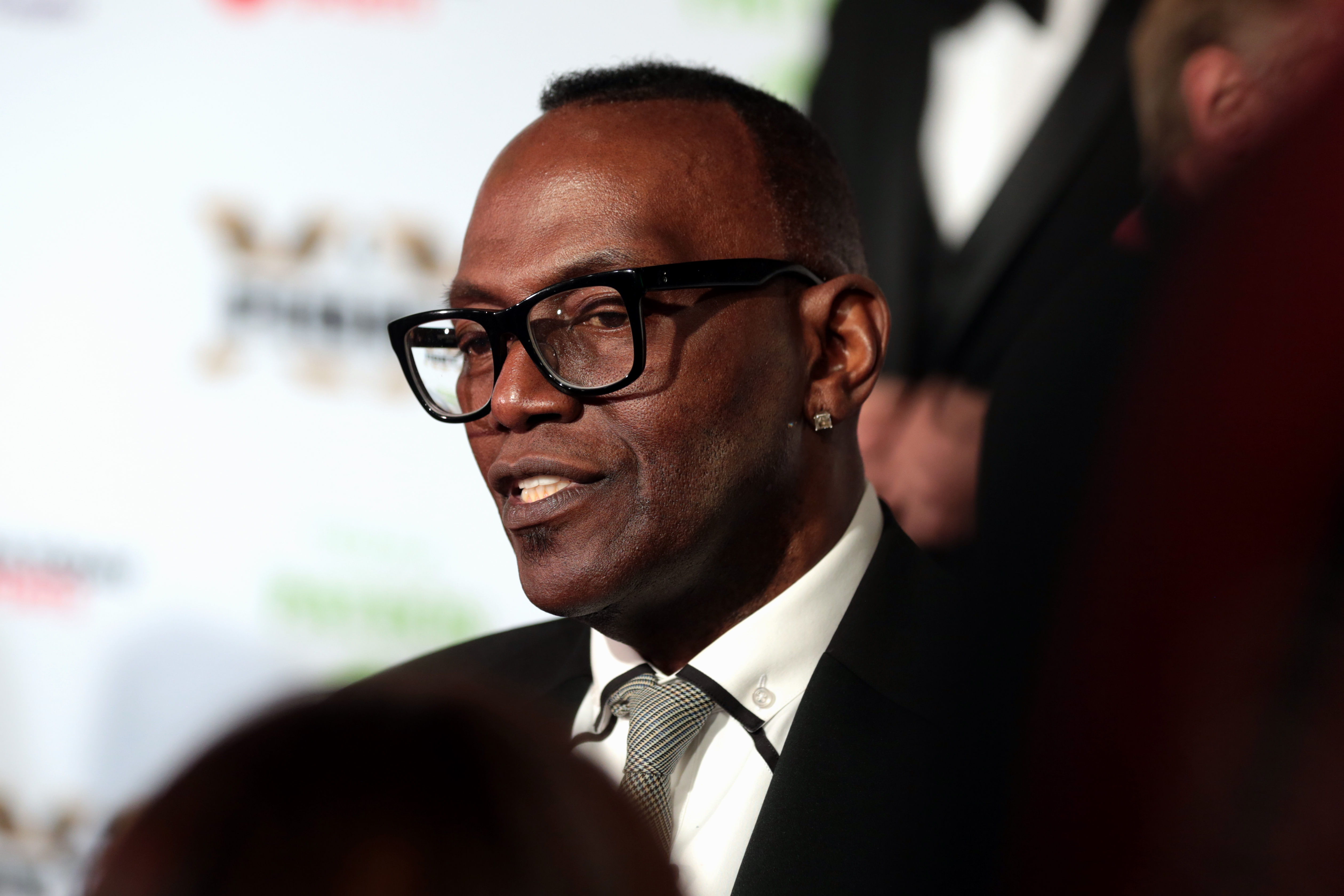The image depicts an African-American male, aged roughly 45 to 50, positioned centrally against a blurred backdrop that appears to feature sponsor names typical of an award show or similar event. The man, who is looking slightly to the left, wears black glasses, a diamond stud earring, and a soul patch. His attire consists of a black jacket paired with a white button-up shirt and a tie. Hints of other figures can be seen around him: a suit and bow tie to his left and a partial view of someone's ear and hair in the background. The overall setting appears to be indoors, possibly during an interview or press conference, with colors including white, orange, green, brown, black, silver, and gray. No text is clearly legible in the image.